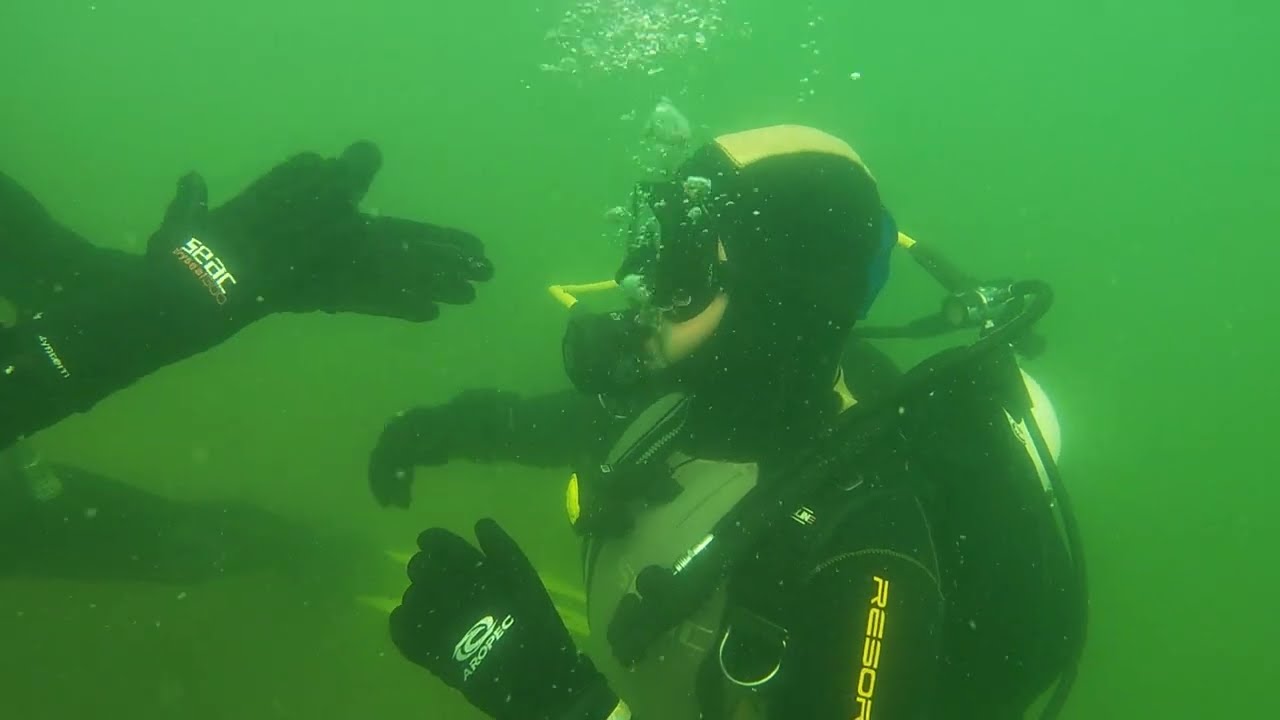The photograph, taken underwater in a murky, green environment, showcases a scuba diver dressed in a black suit with black gloves, a tank on their back, and a mask with goggles. Bright yellow text adorns the side of their suit, though its exact wording is unclear. The diver is surrounded by easily visible bubbles against the green backdrop. In front of the main diver, another person's hands, dressed in black gloves marked with "S.E.A.C" in white, reach forward, likely giving instructions. Additionally, a leg with a flipper, possibly Dayglo orange or yellow, is visible in the background, indicating the presence of a third swimmer moving to the left. The overall scene is characterized by its limited visibility due to the green, seemingly dirty water.